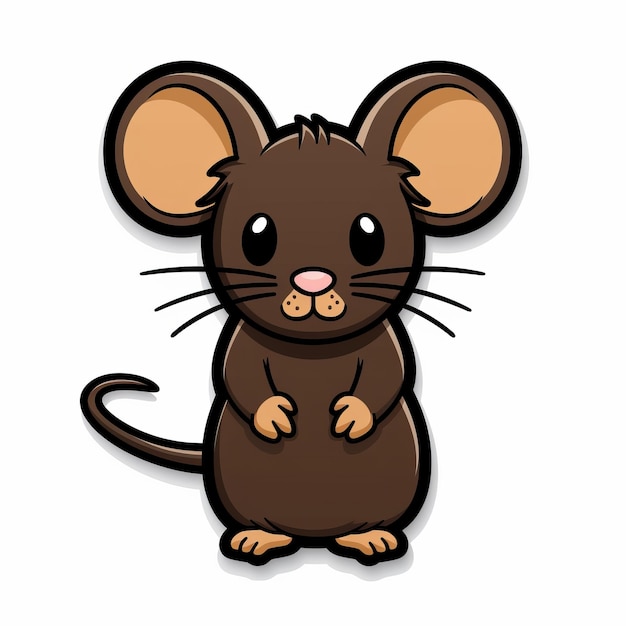This image features a computer-generated graphic of an adorable, cartoon-like mouse centered against a plain white background. The mouse's primary color is dark brown, with black outlines, and it is depicted facing directly at the camera. It has large, round ears with light tan interiors and a cute light pink nose. The mouse's glossy, egg-shaped black eyes are accentuated with small, white highlights. Adding to its charm, the mouse has three long whiskers on either side of its tan muzzle. Its tiny hands and feet are also light tan. The mouse's body is chubby with a wide belly and a small, thin tail that emerges from the bottom left of the image. Additional details include tufts of hair on its head, suggesting a ruffled, playful look.